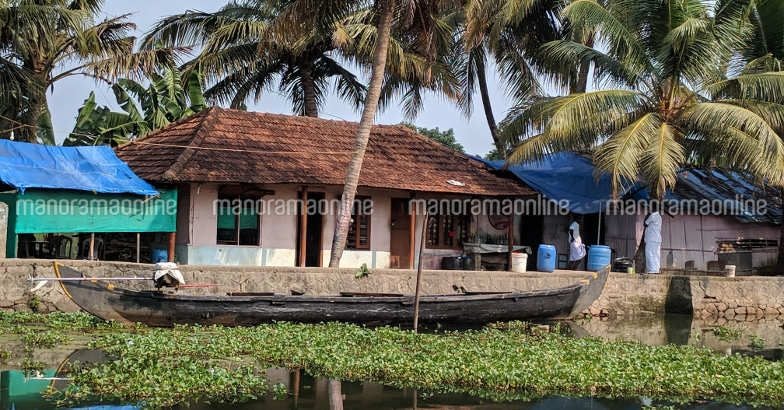In the photograph, a picturesque tropical scene unfolds in what appears to be a small, somewhat run-down village by the water. The main focus is a white single-story vacation house or hut with a brown roof made of a material resembling grass. This central building stands out with its open windows and doors, and it’s flanked by two smaller structures with blue tarp roofs.

The setting is lush, dotted with numerous palm trees that enhance the tropical ambiance. The water in front of the buildings, possibly a shallow part of a river or lake, looks dark and a bit murky, with green foliage floating on the surface. In the center of the water, a black canoe is prominently featured, adding to the serene yet rustic charm of the scene.

Additionally, there are two people, a man and a woman, both dressed in white, standing in front of the main building. Surrounding the buildings are various rain barrels and green plants, contributing to the overall sense of a tropical, possibly third-world, locale. The sky above is clear and blue, suggesting a sunny day in this tranquil, albeit modest, village setting.